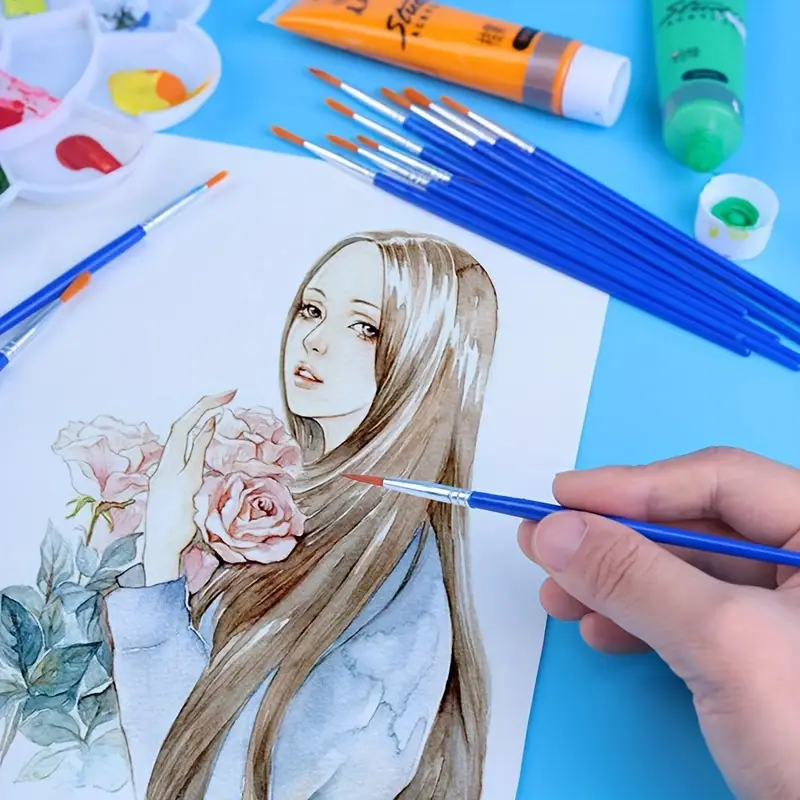The photograph, taken indoors, captures a detailed scene of an artist at work. In the bottom right corner, a hand with lighter skin complexion holds a blue paintbrush between the thumb and index finger, poised over a piece of white paper on a blue table. The paintbrush has a silver front end, and its tip is colored orange. The artwork features a woman with long brown hair flowing down past her waist, wearing a blue long-sleeve shirt. She is facing left but has her head turned to the right, her eyes directed towards the right, and she is holding a bouquet of pink roses. Above the painting, several identical paintbrushes lie scattered, along with an assortment of paint supplies including closed orange, green, yellow, and red squeeze bottles, an open green one, as well as plastic trays with mixed paint to the far left corner. The setting is brightly lit, making details and colors in the scene—light blue, dark blue, light pink, light green, orange, and yellow—stand out vividly. The perspective of the photograph is from above, looking directly down on the artistic process.